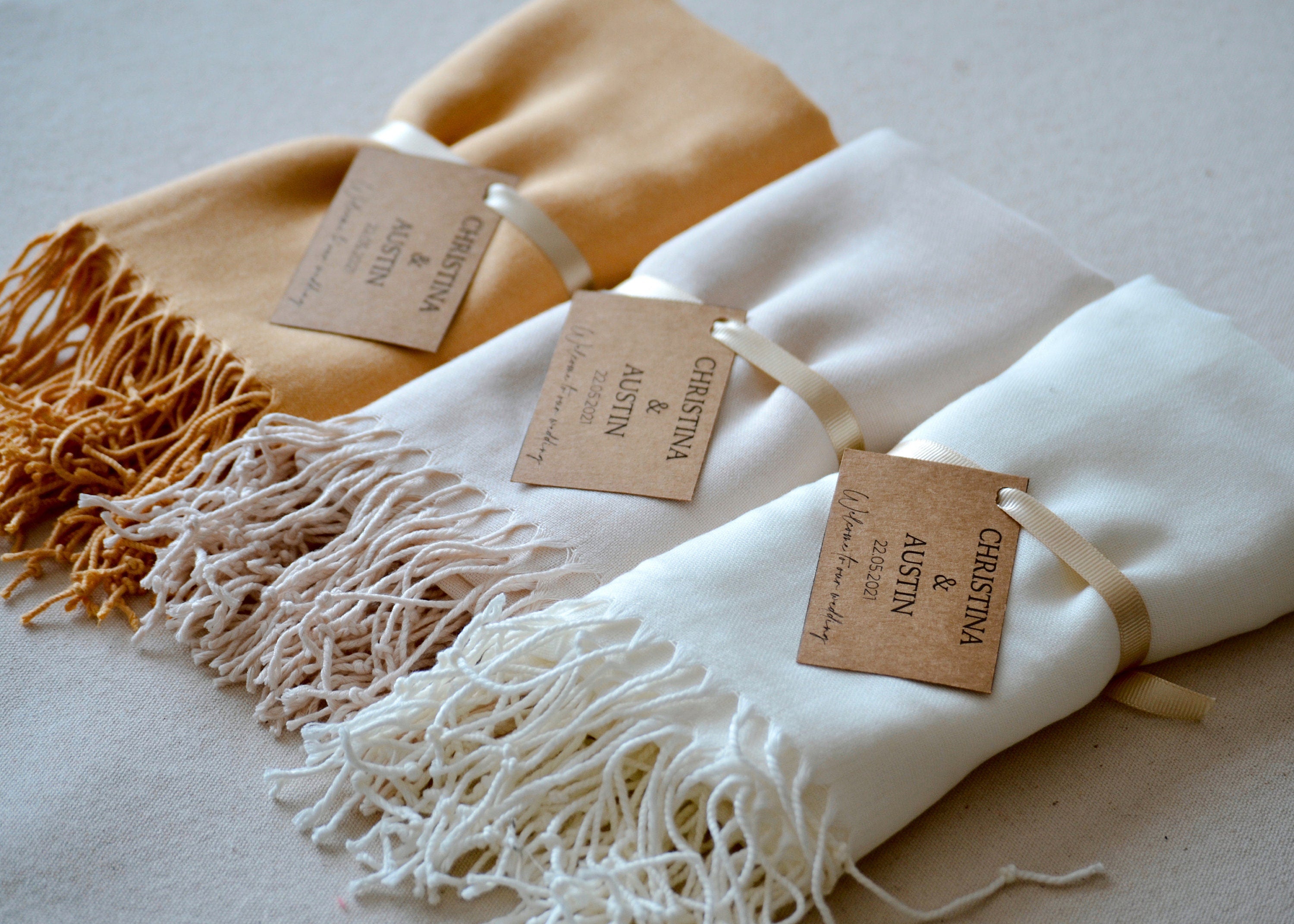The image depicts three high-quality folded cloths with tassels at their edges, arranged from left to right. The cloth on the left is a golden brown color, the middle one is a cream shade, and the one on the right is bright white. Each cloth is meticulously tied with a tan ribbon, attached to which is a rectangular tag that reads "Christina and Austin" along with a date "2-2-0-5-2021," and some smaller, illegible text. These cloths look like they could be special gifts or commemorative items for a significant event, such as a wedding or baby shower hosted by Christina and Austin. The background is a gradient gray, darker on the left side, making the bright fabrics stand out prominently.